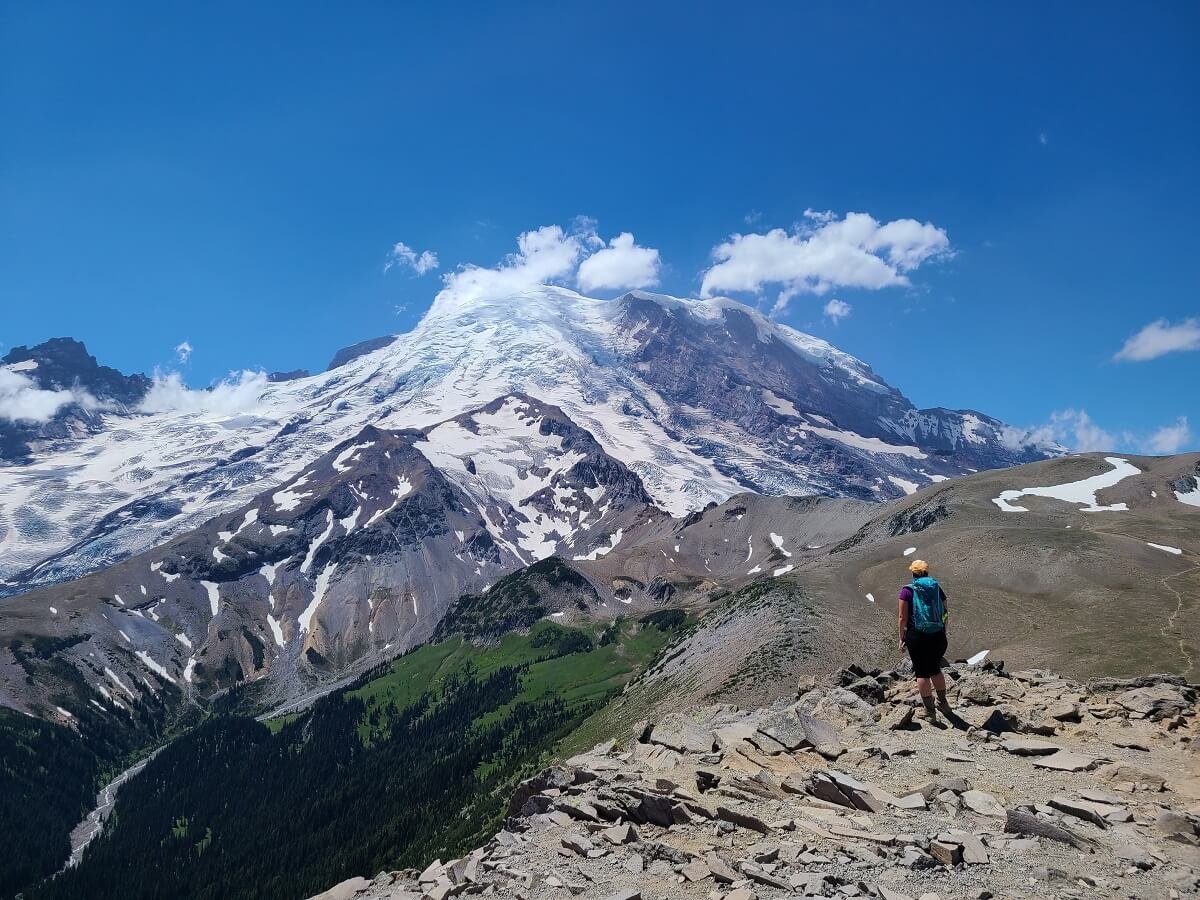In this scenic image of nature, a hiker stands on the rough, rocky terrain on the right side of the photograph. He is dressed in black shorts, a sleeveless dark purple t-shirt, and a yellow baseball cap, with a green backpack slung over his shoulders. The hiker, who has pale skin, gazes out over a breathtaking landscape. To the left of him lies a deep valley filled with lush greenery, trees, and a meandering stream. Multiple peaks rise up from this verdant valley. Further in the distance, a towering mountain dominates the background, its snowy peak gleaming under a clear blue sky dotted with large white clouds. The overall composition captures the serene yet majestic beauty of this mountainous region, showcasing both the hiker's vantage point and the expansive, diverse terrain that spreads out before him.